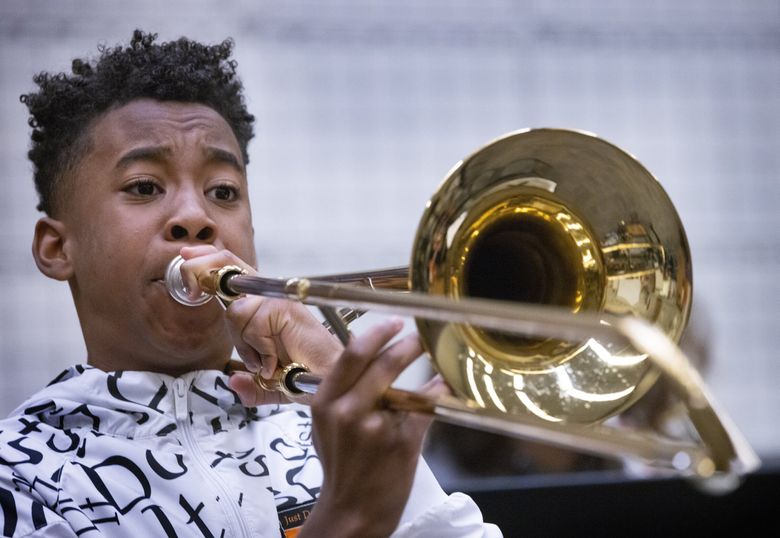In this captivating image, a young Black American boy with rich melanated skin is seen passionately playing a trumpet. His facial expression reveals the intense effort required to play the instrument, with his cheeks puffed out and deep concentration lines creasing his forehead. His hair, a type 4c with tightly coiled curls, crowns his head. He wears a striking black and white jacket with a hood and long sleeves, adding a stylish touch to his determined stance. The background is a minimalist blend of white and black, which serves to highlight the boy and his trumpet in vivid detail.